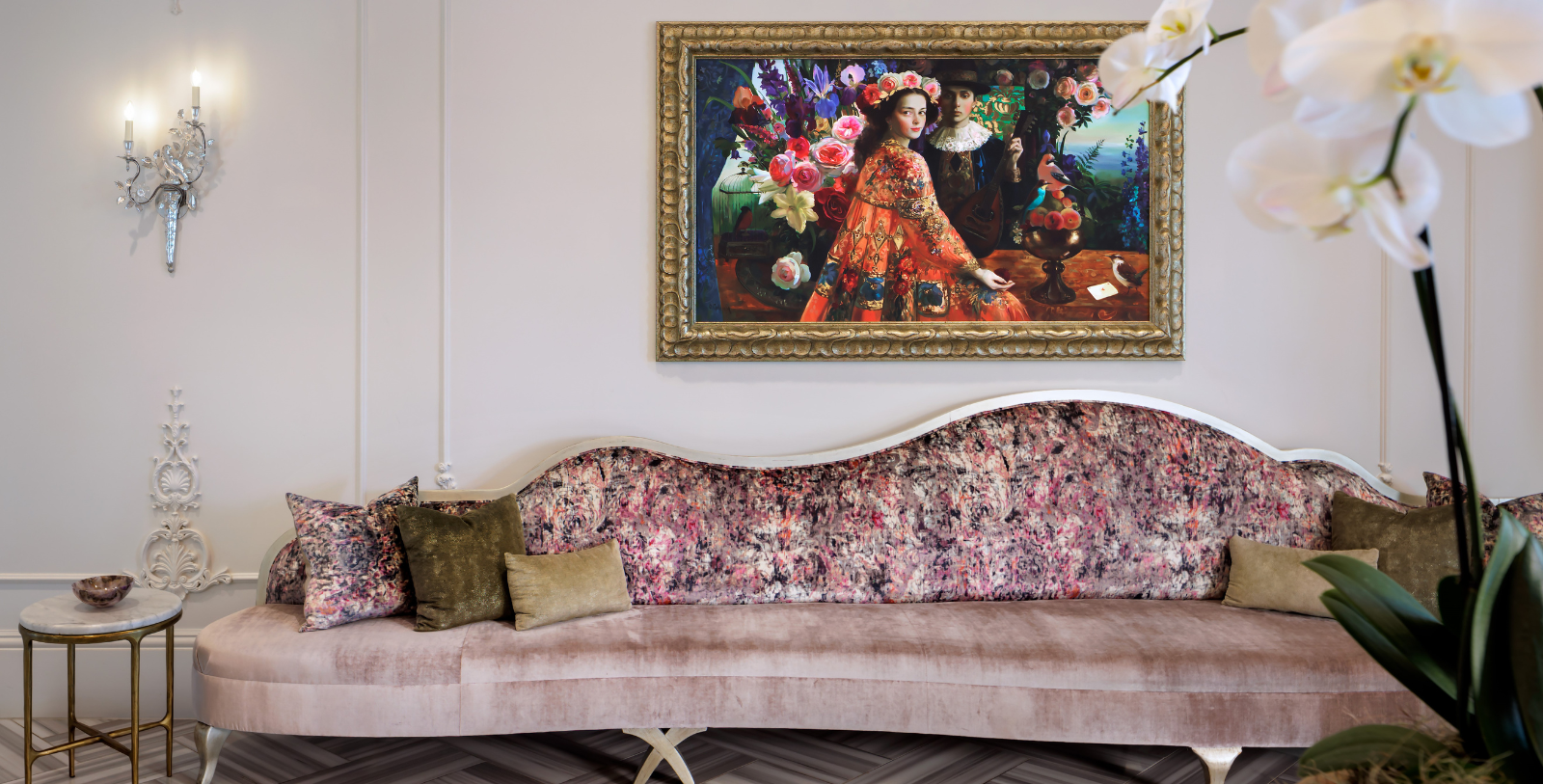In the image, there is an antique-style, very long couch with a velvet texture. The couch has a light pink seat cushion and a floral-patterned velvety back in shades of pink, light red, black, and white, giving it a speckled appearance as if paint was splattered on it. There are four throw pillows: two are tan, one is olive green, and one matches the floral pattern of the couch’s back.

To the left of the couch is a gold-painted end table with a marble top, holding a small dish. The white walls are trimmed with white, and to the left side, there is a silver sconce with two taper candles, likely LED, casting a soft light. A potted plant with green leaves and white petals sits nearby.

Above the couch hangs a large painting depicting a couple dressed extravagantly, the woman adorned with a flower headdress, surrounded by flowers and a scenic horizon in the background. The scene provides a beautiful, nature-infused backdrop that complements the classic elegance of the sofa.